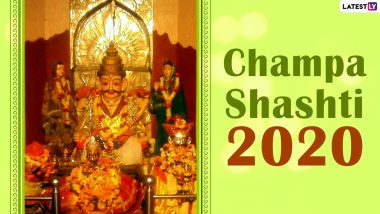This full-color promotional image is divided into two vertical panels. The right panel features a lime green background with lighter areas and contains the text "Champa Shasti 2020," where "Champa Shasti" appears in dark green and "2020" in red. In the upper right-hand corner of this panel, the word "latest" is written in black. The left panel displays an image of what appears to be a group of Hindu religious statues, with details suggesting they might be from India or Pakistan. The statues, five in total, are depicted with extremely faded colors and poor lighting. They appear to be sitting on a gold throne, showcasing an ornate design with dominant hues of yellow and red. The photograph overall is poorly executed in terms of color and lighting.